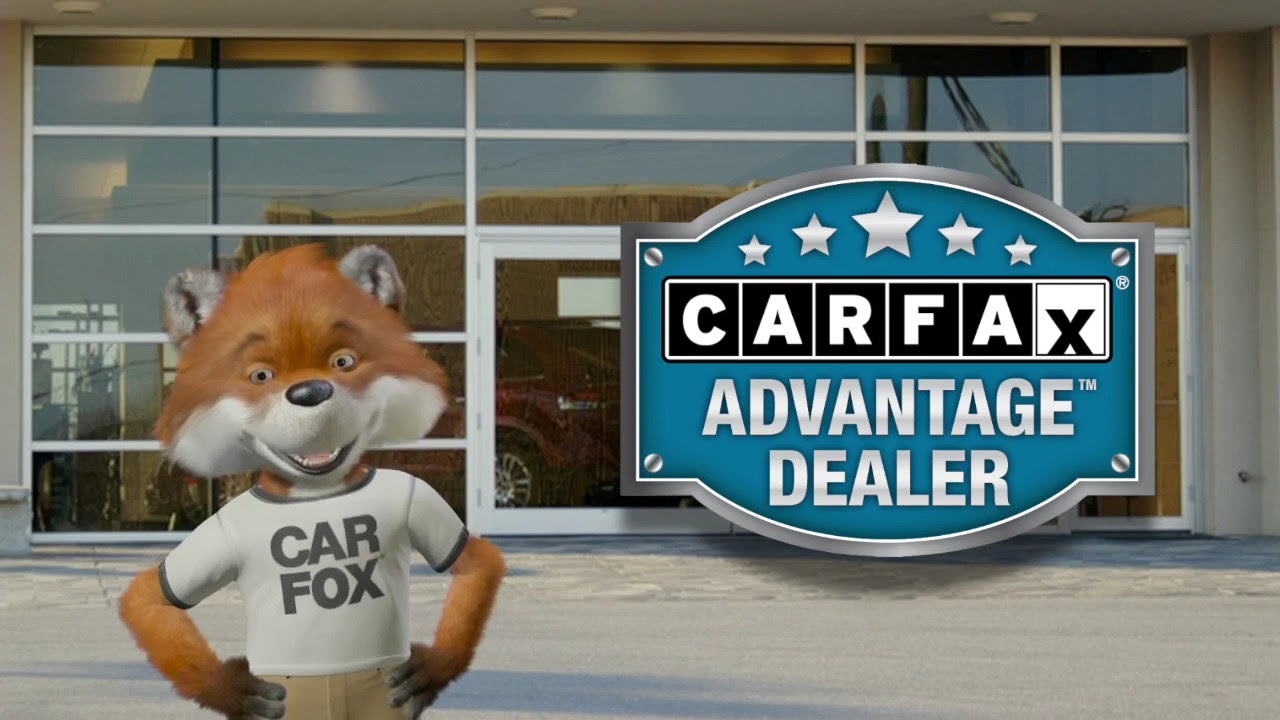The image appears to be a promotional still, possibly from a car commercial or print advertisement, depicting an automotive dealership. The backdrop showcases a large storefront with extensive glass windows framed in white, providing a view inside where several cars are parked. On the left side of the frame, a 3D illustration of a mascot— a cartoon fox— stands with its hands on its hips, wearing a white t-shirt emblazoned with "Car Fox" in gray or black text. To the right of the fox, a prominent emblem features the Carfax logo in a blue bubble, accompanied by the text "Advantage Dealer." The ground in front of the storefront is a whitish cement color, adding to the professional ambiance of the dealership setting.